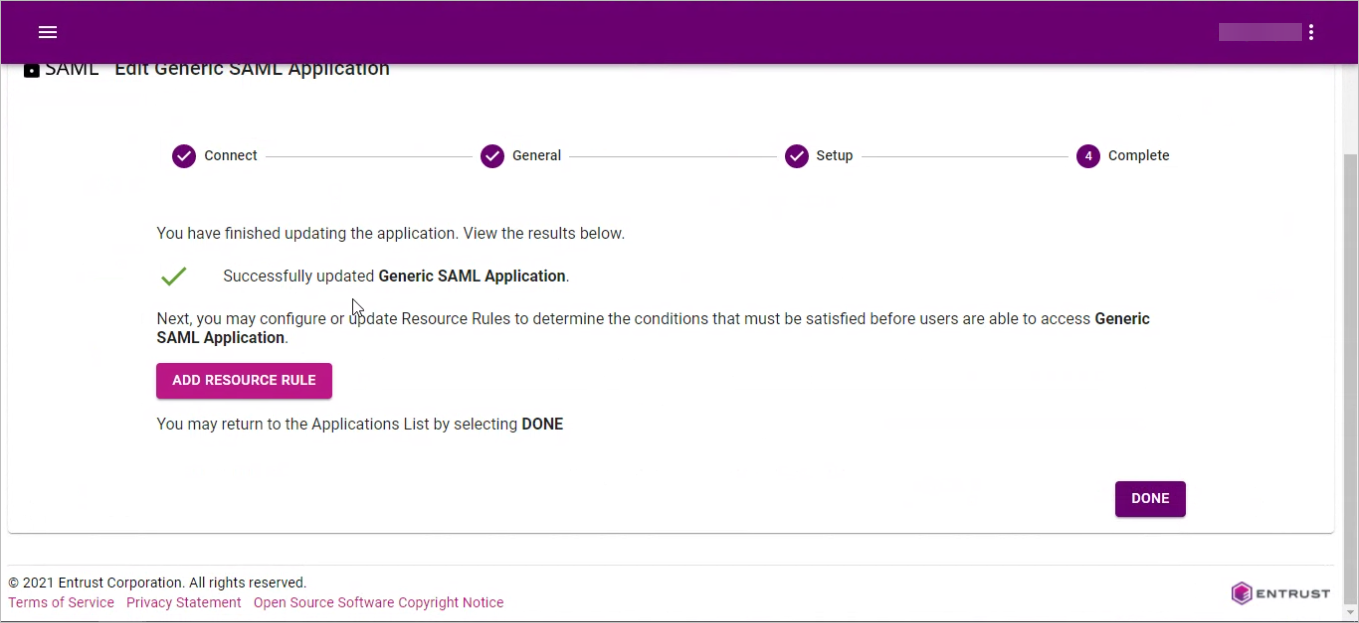The image features a user interface with a purple top bar. On the upper left corner of this bar, there are three white horizontal lines. On the right, there is a lighter purple box. Below the bar, a white page is visible with the header "SAML - Edit Generic SAML Application." Below the header, there's a progress line with several labeled checkmarks: "Connect," "General," "Setup," and a fourth step "Complete" without a checkmark.

The page also displays a message: "You have finished updating the application. View the results below," followed by a green checkmark and the text "Successfully updated Generic SAML Application." Below this, in bold text, it reads, "Next, you may configure or update resource rules to determine the conditions that must be satisfied before users are able to access Generic SAML Application." 

A purple-pink button labeled "Add Resource Rule" in white text is situated underneath. Another message reads, "You may return to the applications list by selecting Done," with a purple button labeled "Done" located at the bottom right of the page. In the bottom left corner, the footer displays the text "© 2021 InTrust Corporation. All rights reserved," followed by links to "Terms of Service," "Privacy Statement," "Open Source Software Copyright Notice." Finally, the bottom right corner features the "InTrust" logo alongside its trademark.